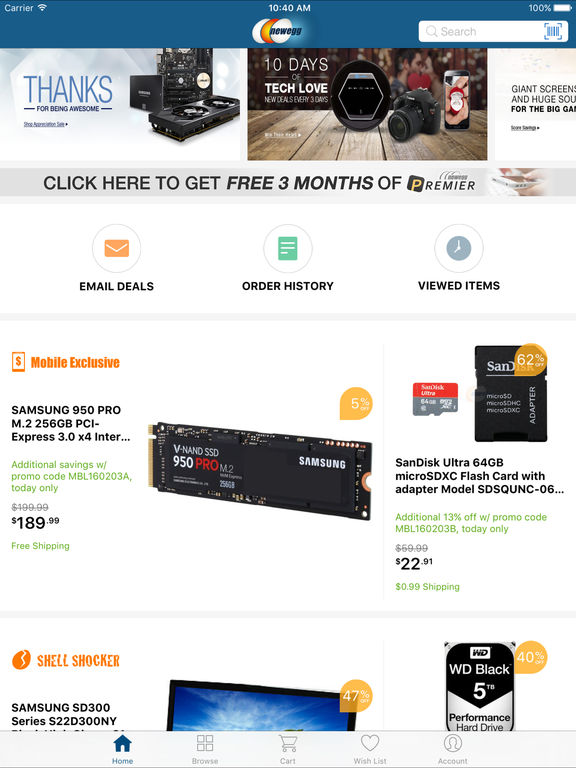**Detailed Advertisement Image Description:**

The image resembles a digital advertisement with several distinct sections and elements.

1. **Header Section**:
   - **Background**: Blue.
   - **Top Left**: "Carrier" followed by a Wi-Fi logo.
   - **Center**: "10:40 AM" in white font.
   - **Middle**: A logo featuring red, white, and black text.
   - **Right**: 
     - Battery icon at 100% charge.
     - Squarish box with three lines resembling a menu icon.
     - White square containing a magnifying glass icon with the word "search" next to it.

2. **Main Body**:
   - **Top Section**: Black box with blue text saying "Thanks" and black text saying "for being awesome". To the right, it states "10 days of" in black and "tech love" in white with a camera icon resembling a phone to the right, featuring an image of Santa Claus.
   - **Middle Right Section**: 
     - Text that reads "Giant screen and huge sound for the big game".
     - Below this, in black font: "Click here to get free three months of Premiere".
     - White background featuring icons for different sections: 
       - Orange envelope and gray circle for "email deals".
       - Green box with white lines in a gray circle for "order history".
       - Gray clock icon for "viewed items".
       - Mobile exclusive section with an orange underline and a text "Samsung 950 Pro M.2, 256 GB PCI, Express 3.0 x4". Below, in green font: "Additional savings W/ promo code MBL160203A, today only". Previous price in gray ($199.99) and current price in green ($189.99) with "free shipping in green". Above the price, there's an orange placeholder with "5".
   - **Product Details**:
     - Black square with "Samsung" in white text followed by "V hand SSD". Below, in white text: "950 Pro" and "M.2" in gray. 
     - SanDisk product details: 
       - Orange circle showing "62%" discount.
       - Black disc icon with gray lettering below.
       - Red and gray squares with SanDisk Ultra 64GB Micro SDXC Flash card, model SDSQUNC-06. Below in green font: "Additional 13% off with promo code MBL160203B, today only". Previous price in gray ($59.99) and current price ($22.91) with "99 cents shipping in green".
   - **Shell Shocker Section**:
     - Orange cracked egg icon and text: "Shell Shocker".
     - Samsung product detail: "Samsung SD300 series, S22D300NY". Representation of a half screen with 47% discount in an orange circle.
     - Black square with a black triangle and white square saying "WD", followed by "WD Black 5". Orange circle with 40% discount and white background text: "Performance Hard Drive".

3. **Footer Navigation**:
   - Icons with text: 
     - "Home" with a blue house icon.
     - "Browse" with four squares.
     - "Cart" showing an image of a cart.
     - "Wishlist" with a gray heart icon.
     - "Account" with a face icon in a circle.

This complex image is packed with various promotional offers, product details, and interactive elements designed to engage the viewer with vibrant colors and detailed information.